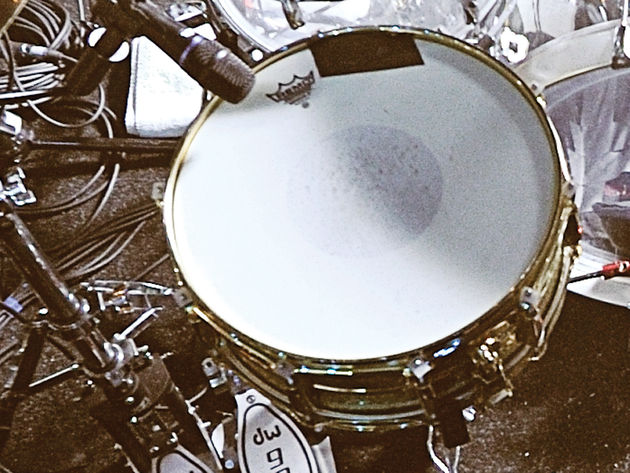This top-down photograph features a primary focus on a large, circular drum situated slightly off-center towards the top right. The drum, which is silver around the edges, features a white drum skin adorned with a black crown logo labeled "Remo" at the top. The image is predominantly monochromatic, composed of black, white, and shades of gray, with minimal coloration. 

In the upper left corner, a black microphone on a black tripod stand leans towards the center of the drum, suggesting it is positioned to record. Adjacent to the microphone are numerous black cords and cables strewn across the ground. The rough, dark gray flooring, possibly asphalt, indicates an outdoor or rugged indoor setting such as a garage. 

Additional drum set components are visible in the background, both at the top and to the right side of the image. In the bottom left-hand corner, part of a microphone stand and potentially another drum are present. Above and to the left of the cords, a white object that appears to be a towel can be seen. The overall scene is one of a musical setup, showcasing equipment amidst a stark, color-limited environment.